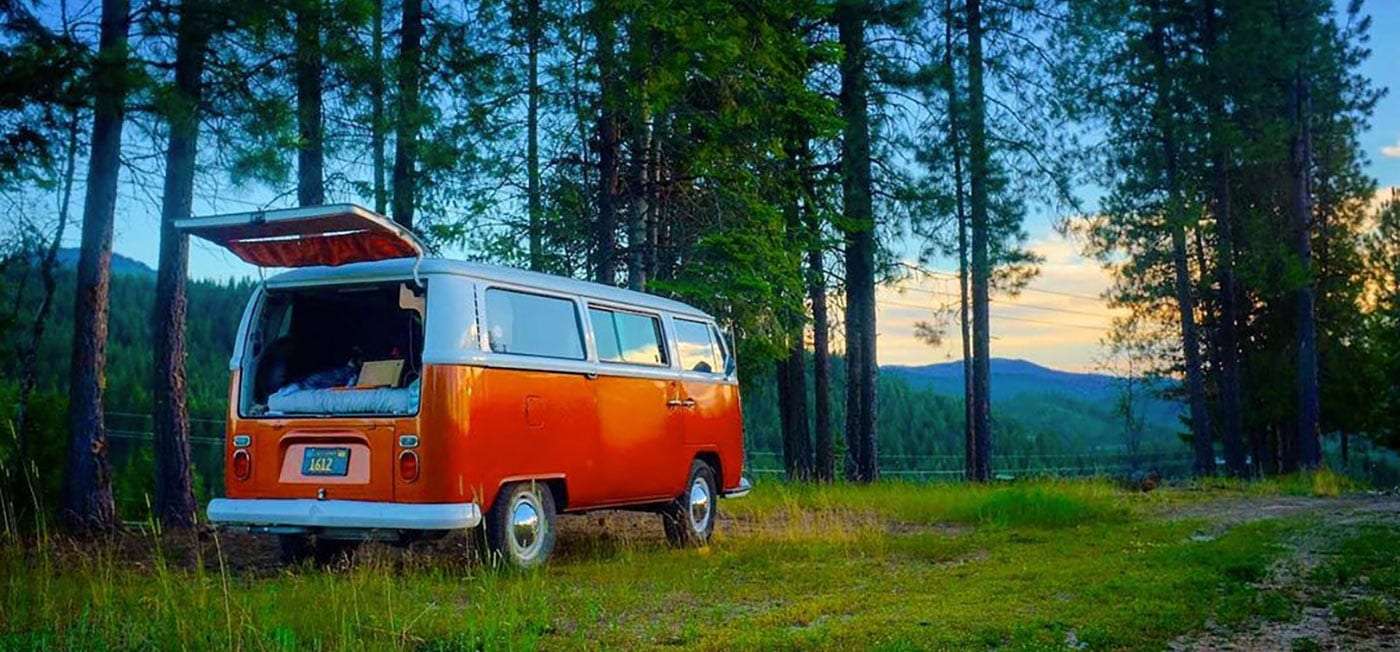In this wide-angle shot of a serene California wilderness, a vintage orange-and-white VW camper van sits on the left side of a grassy parking area surrounded by sparse pine trees. This picturesque campsite features a lifted rear hatch revealing a cozy bed setup inside. The van's classic charm is accentuated by its chrome hubcaps and silver bumper, while the blue California license plate confirms its location. The scene is bathed in the golden hues of late afternoon, with a backdrop of low, tree-covered mountains and a stunning sky dotted with blue, pink, and orange clouds. In the foreground, a gravel path weaves through the grass, adding to the idyllic atmosphere. The van has three visible windows on the passenger side, along with its distinctive two-tone paint job and red taillights. This beautifully captures the essence of a tranquil camping experience in the California mountains.